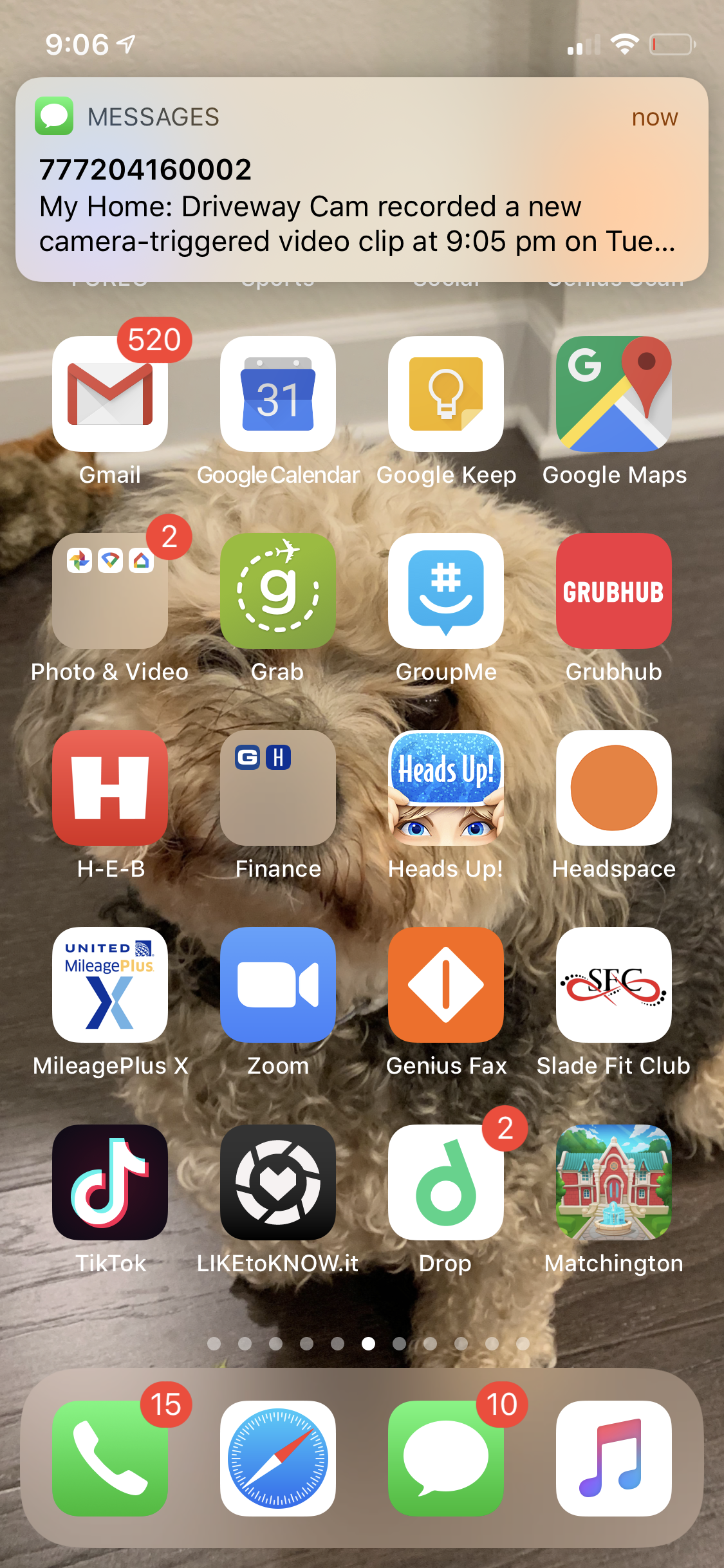This image is a screenshot from a cell phone, showcasing a layered composition with various visual elements. The background features a cozy scene of a dog with a curly, multi-colored coat consisting of white and darker brown shades. The dog's fluffy, long-haired floppy ears, black eyes, and stubby nose are prominently visible against a white wall and dark wood floor backdrop.

Overlaying the dog background are several rows of small squares, arranged in a grid pattern. At the top of the screen, the status bar shows "906" with a signal strength indicator on the top left, while on the top right, icons include two small vertical lines, three stacked horizontal lines, and a battery symbol.

Below the status bar is a notification rectangle that reads "MESSAGES NOW," followed by a detailed alert: "MY HOME DRIVEWAY GANG RECORDED A NEW CAMERA TRIGGER VIDEO CLIP AT 9:05 PM ON TUESDAY." Further down, the interface displays five rows of four colored squares, each symbol representing different applications or functions.

The lower section of the screen features a semi-transparent rectangle containing four distinct symbols, topped by a row of dots, likely indicating pagination or additional content screens. The overall screenshot provides a detailed glimpse into the user's mobile interface, combining functional elements with a visually appealing background.